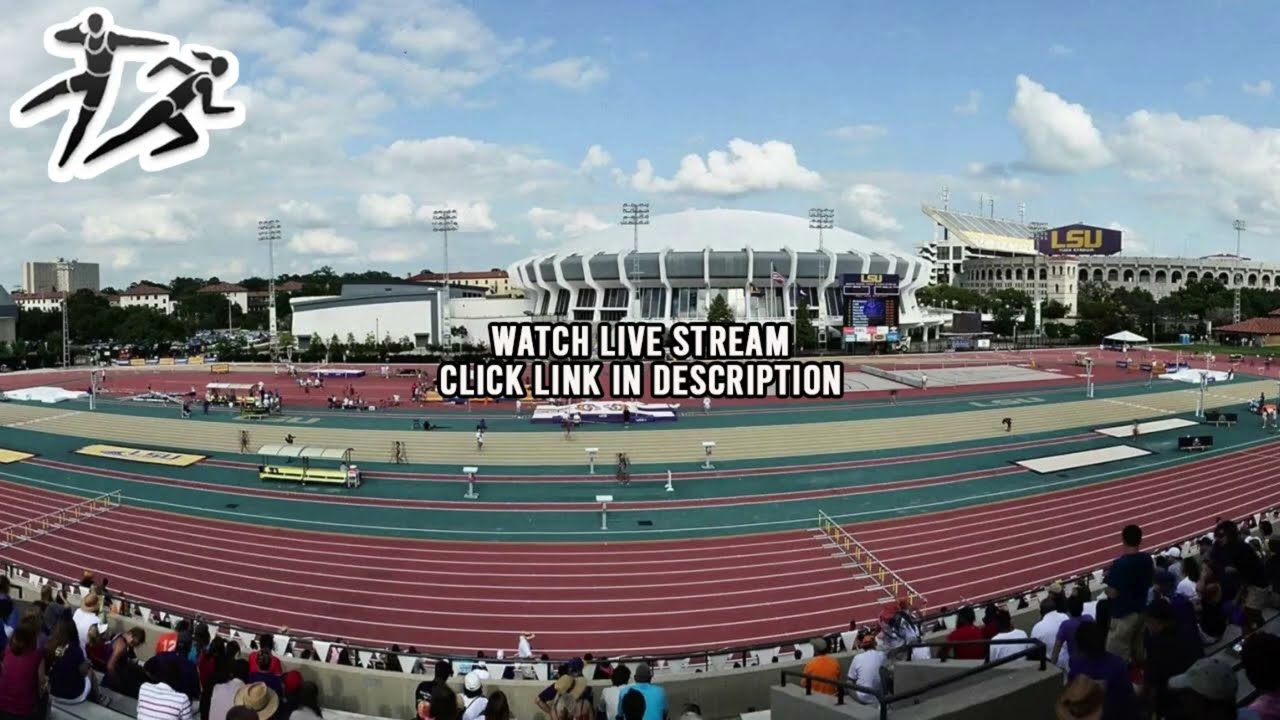This detailed photograph captures an outdoor track and field setup at Louisiana State University (LSU) in Baton Rouge, seen from the upper stadium stands. The viewer's perspective is from high above, looking down over the vividly colored athletic field. The primary focus is the red track with clear white lane markings, notably set up for a hurdles race with two sets of hurdles directly in front. The infield is a rich green, structured for various field events, and transitions into another track section with a couple of red stripes, followed by a light yellow strip and additional green areas, ultimately leading to a large, open red field.

Spectators are sprinkled in the stands below, highlighting the community's involvement in these athletic events. The stadium features metal barricades, and a distinctly visible LSU sign marks one of the circular buildings in the backdrop, likely part of the college campus's sports complex. The bright blue sky is dappled with white, fluffy clouds, suggesting pleasant, albeit potentially cloudy weather conditions.

In the image’s center, white script with a black outline reads, "Watch live stream. Click link in description." In the upper-left corner, there are digital icons of two athletes: one appears to be throwing a discus, and the other is a female runner, which adds a dynamic touch to this collegiate sports scene. The overall ambiance suggests a day bustling with track and field events, perfect for a live broadcast.